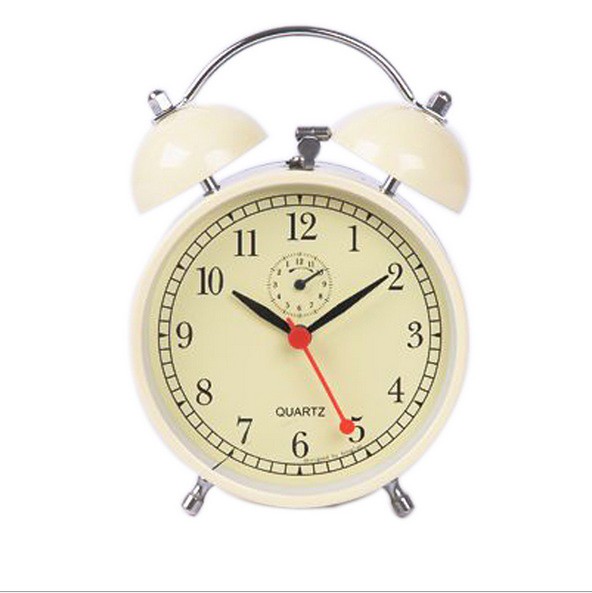The image depicts a classic, vintage-style alarm clock with a distinctive design. The clock features a 3D circular body and stands on two metal prongs, serving as feet. It boasts a creamy yellow face adorned with traditional numerical markings, with the number 12 at the top and the number 6 at the bottom. The main hands of the clock, the hour and minute hands, are black, while the second hand is thinner and red with a small circle at its end. Above the number 6, the word "QUARTZ" is prominently displayed.

At the top of the clock, two beige or cream-colored bells are situated, resembling ears, and are connected by a small curved metal bar secured with screws. These bells are part of the clock's alarm mechanism. The clock's face is bordered with tiny squares, adding to its antique aesthetic, and features an additional smaller circle under the number 12, resembling a secondary clock or timer, with a small hand pointing from the number 2 to the number 10. This intricate design combines both functionality and a touch of nostalgic charm.